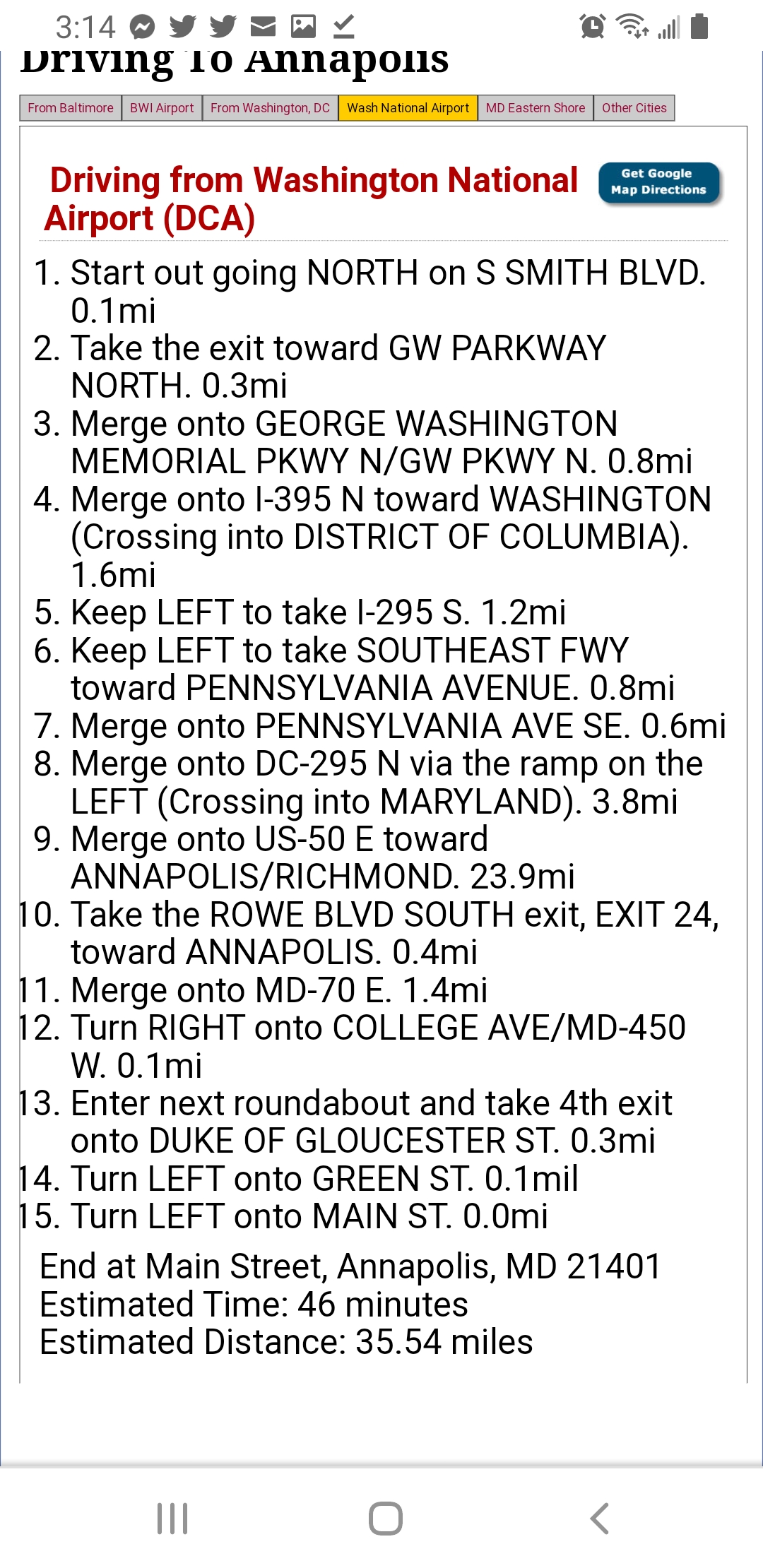The image showcases a detailed driving directions interface, typical of what one might find using a navigation app or a search engine like Google. At the top, in bold black lettering, it declares "Driving to Annapolis." Directly below, set against a white background, the starting point is indicated in red: "Driving from Washington National Airport (DCA)."

The directions provided are numbered and written in black text, offering a step-by-step guide to Annapolis:
1. **Start out going north on South Smith Boulevard** for 0.1 miles.
2. **Take the exit toward GW Parkway North** for 0.3 miles.
3. **Merge onto George Washington Memorial Parkway North (GW Parkway North)** for 0.8 miles.
4. **Merge onto I-395 North towards Washington**, crossing into the District of Columbia, for 1.6 miles.
5. **Keep left to take I-295 South** for 1.2 miles.
6. **Keep left to take the Southwest Freeway toward Pennsylvania Avenue** for 0.8 miles.
7. **Merge onto Pennsylvania Avenue Southeast** for 0.6 miles.
8. **Merge onto DC-295 North via the ramp on the left**, crossing into Maryland, for 3.8 miles.
9. **Merge onto US-50 East towards Annapolis/Richmond** for 23.9 miles.
10. **Take the Rowe Boulevard South exit (Exit 24) towards Annapolis** for 0.4 miles.
11. **Merge onto MD-70 East** for 1.4 miles.
12. **Turn right onto College Avenue (MD-450 West)** for 0.1 miles.
13. **Enter the next roundabout and take the fourth exit onto Duke of Gloucester Street** for 0.3 miles.
14. **Turn left onto Green Street** for 0.1 miles.
15. **Turn left onto Main Street**, arriving at your destination: Main Street, Annapolis, MD 21401.

The estimated travel time is 46 minutes, covering an estimated distance of 35.54 miles.